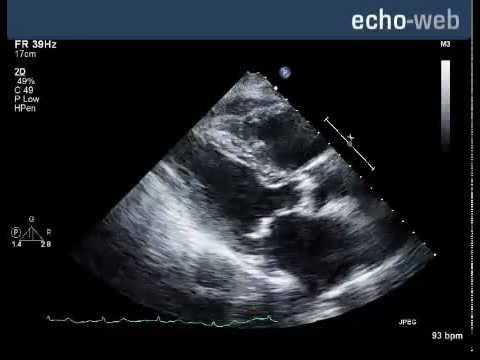This detailed ultrasound image is oriented in landscape mode and prominently features the title "Echo/Web" at the top right, with "echo" in white and "/web" in darker gray. The image is primarily black and white, resembling an X-ray or sonogram, and depicts a vague, cone-shaped outline that suggests an ultrasound of a baby in a womb, although the silhouette is not distinctly visible. Positioned on the left side of the image are several technical details: "FR 39Hz", "17CM", "2D", "49%", "C 49", "P low", and "H pen." Centrally on the bottom right, the image shows a heart rate of "93 BPM." Additionally, there is a triangular diagram on the center left side of the image, the exact details of which remain unclear. Just below the center on the left side, there is a "P" enclosed in a circle with the number "14" beneath it. Overall, the mysterious and somewhat indistinct outline, combined with detailed technical specifications, suggests the ultrasound captures imagery of a baby before birth.